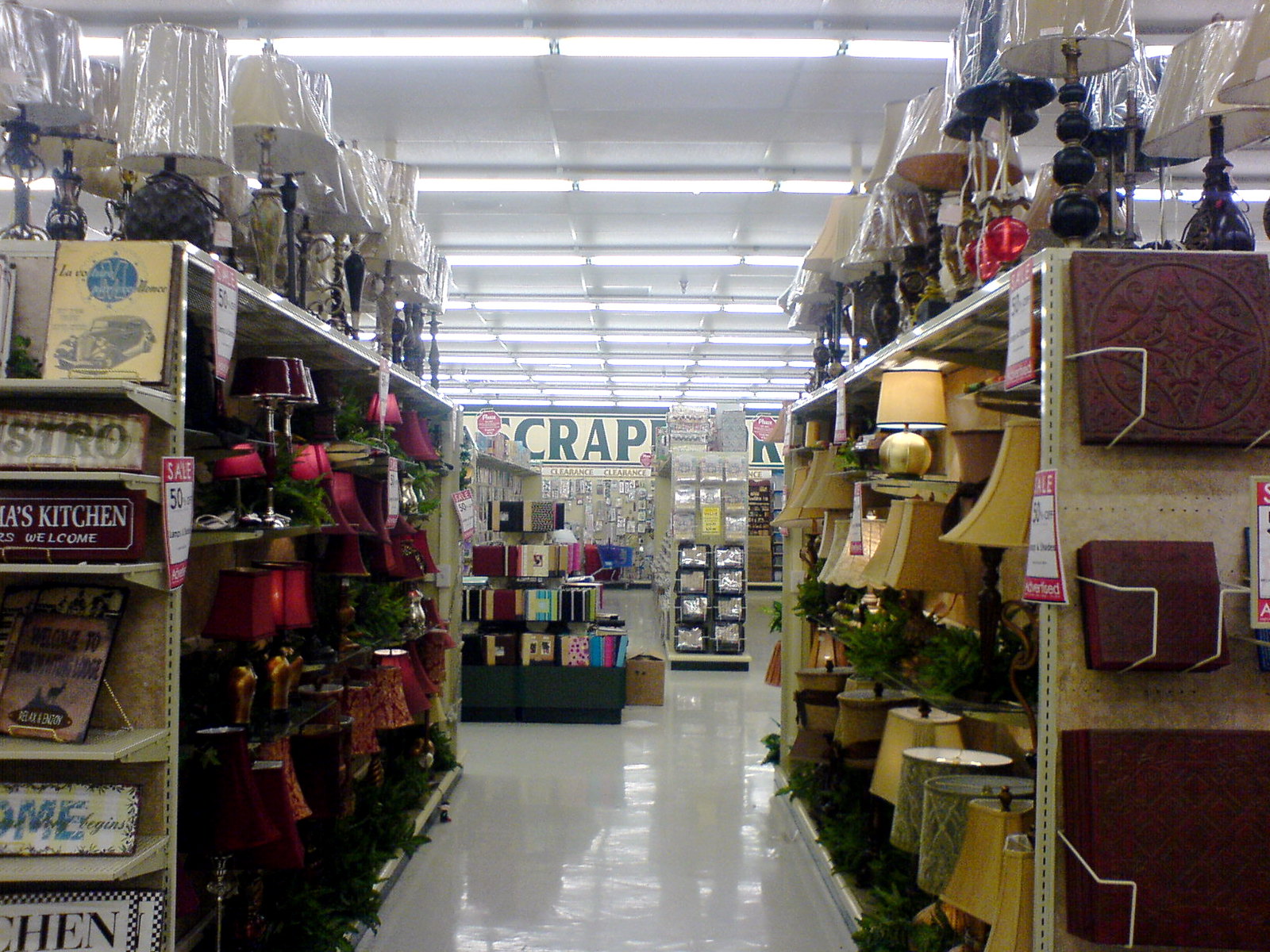This image depicts the view down the central aisle of a large variety store, reminiscent of a big box retailer. Prominently situated in the center is a sign that spells out "S-C-R-A-P," indicating a section dedicated to scrapbooking supplies. The aisle is lined with a diverse array of items, dominated by a selection of lighting products, including both table lamps and floor lamps. Various types of stationery are also visible, alongside an assortment of other merchandise that extends into the distance. The store’s expansive layout is highlighted by the long rows of shelving and the extensive lighting overhead, which stretches far beyond the visible racks. At the end of the aisles, additional signage, logos, and knickknacks hint at the store's vast inventory. The high ceiling adds to the impression that this store offers an extensive variety of goods, catering to a wide range of shopping needs.